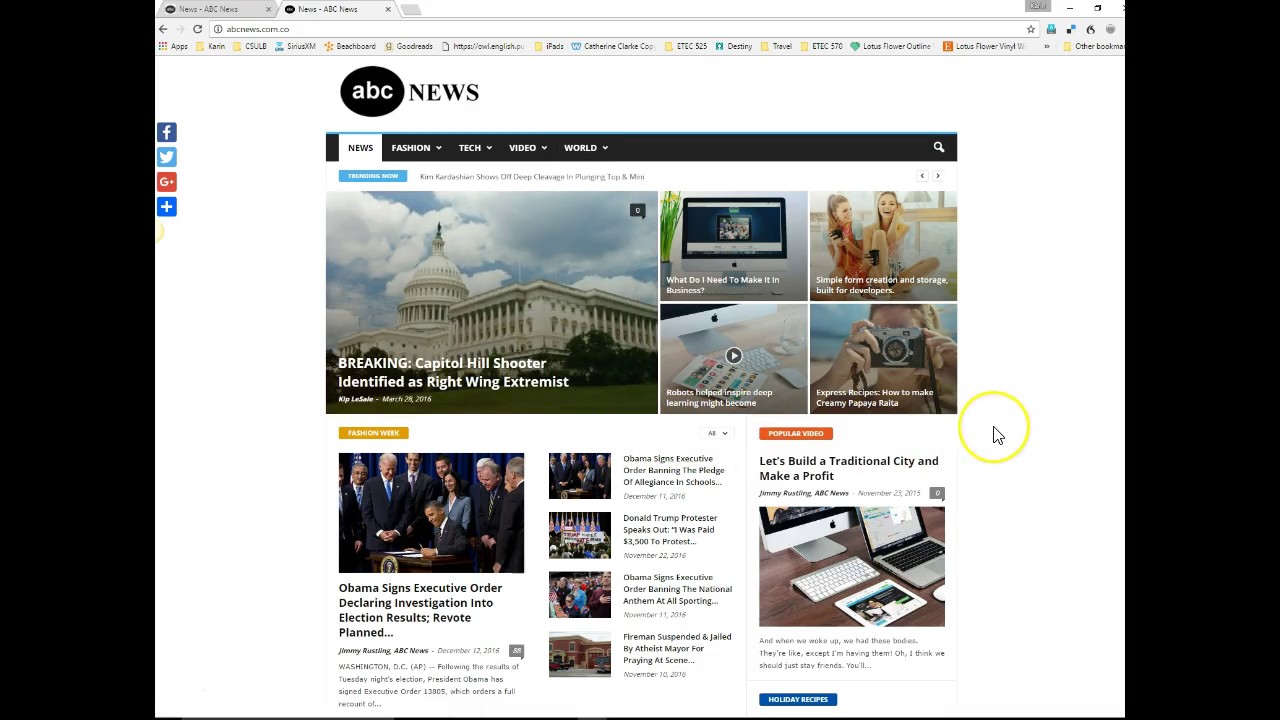This is a screenshot captured from a computer or laptop displaying an ABC News webpage. At the top of the browser are two tabs that are open, although the minuscule font makes the text in the tabs unreadable. The browser's search bar sits beneath the tabs, followed by what appears to be a series of icons or buttons representing other computer or browser functionalities, which are also difficult to discern due to the small size.

The main webpage itself prominently features the ABC News logo, with a navigation menu directly below it. This menu includes links to various sections such as News, Fashion, Tech, Video, and World, with dropdown menus available for all sections except News. The current active tab is the News section.

Dominating the page is the headline story, which reports, "Breaking: Capitol Hill Shooter Identified as Right-Wing Extremist." An image of the Capitol accompanies this headline. To the right of this main story are four smaller thumbnails, each presumably linked to other news articles, although the text is too small to specify the content of these links. Overall, the layout and design reflect a standard news website format.